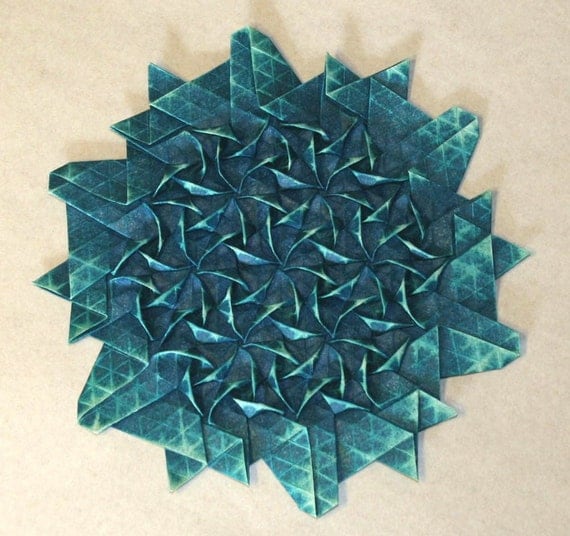This photograph features a star-shaped decorative object resting on a flat, tan-colored surface, which might be stone but is difficult to identify definitively. The surface resembles something sandy or stone-like, adding a natural texture to the scene. The object itself, reminiscent of a blend between a plant and origami, exhibits a complex, geometric design with varying shades of green, ranging from light to dark hues.

The outer edges of the decoration consist of pointed juts or small triangles, lending it a starburst or sunburst appearance. Within this border, the decoration features layers of leaf-like structures adorned with intricate spines and lines, presenting a mix of white, yellow, and green colors. The inner part includes more sharp, thin, light-green blades arranged around small circular elements, providing a detailed, almost botanical aesthetic. Shadows cast by the object enhance its three-dimensional quality, indicating good illumination and contributing depth to the image.